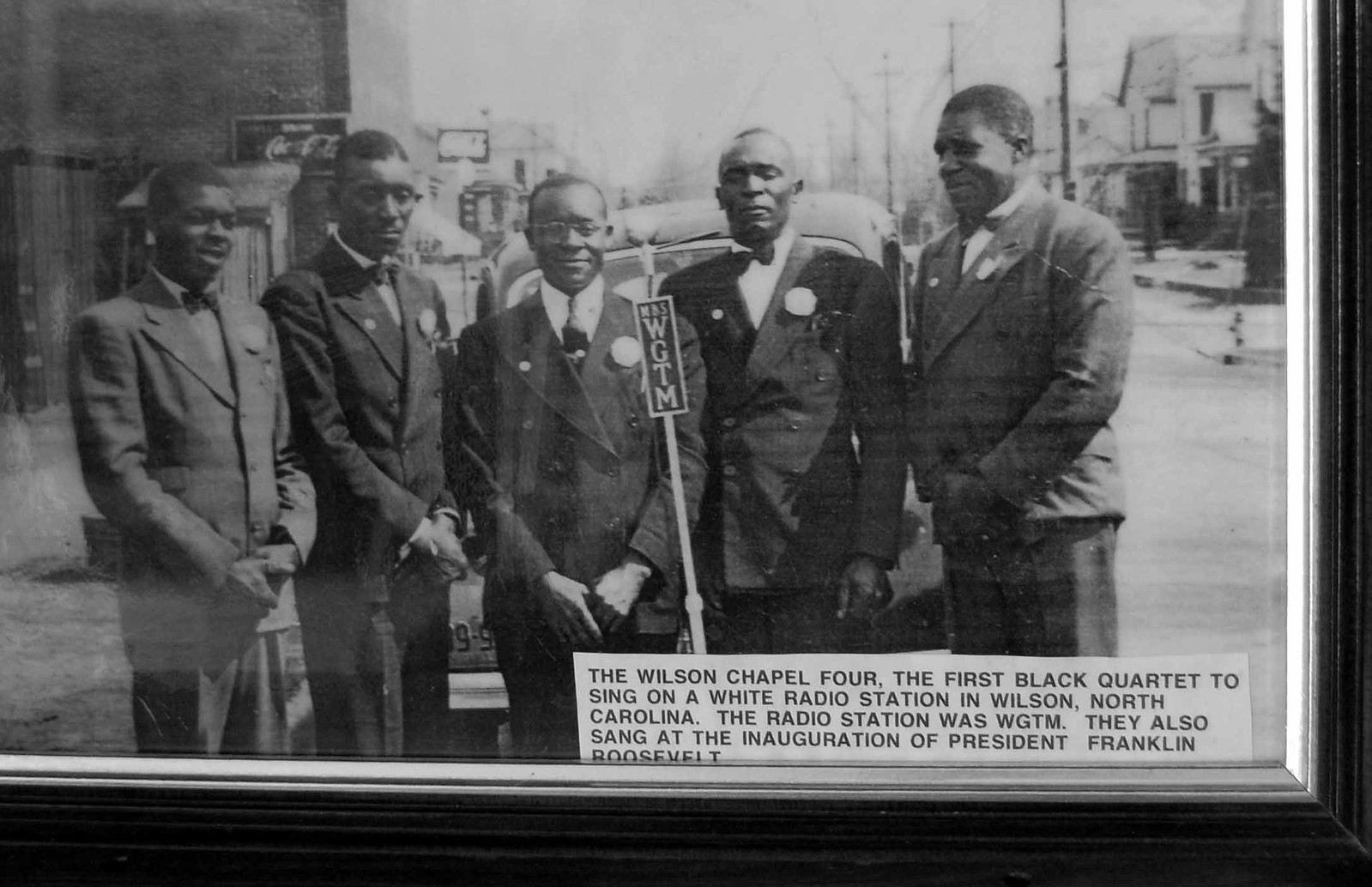This is a black and white photograph capturing five well-dressed Black gentlemen, each donning black suit jackets and shirts. Four of the men are adorned with bow ties, while one sports a conventional tie, and all feature either a button or boutonniere on their lapel. The gentlemen, all of whom have short black hair, stand outdoors on a street, evidenced by the car and some houses in the background. Prominently featured is a Coca-Cola sign and a microphone marked for WGTM radio station. The photo captures the group known as the Wilson Chapter Four, the first Black quartet to perform on a white radio station in Wilson, North Carolina. Notably, they were also honored to sing at the inauguration of President Franklin Roosevelt.